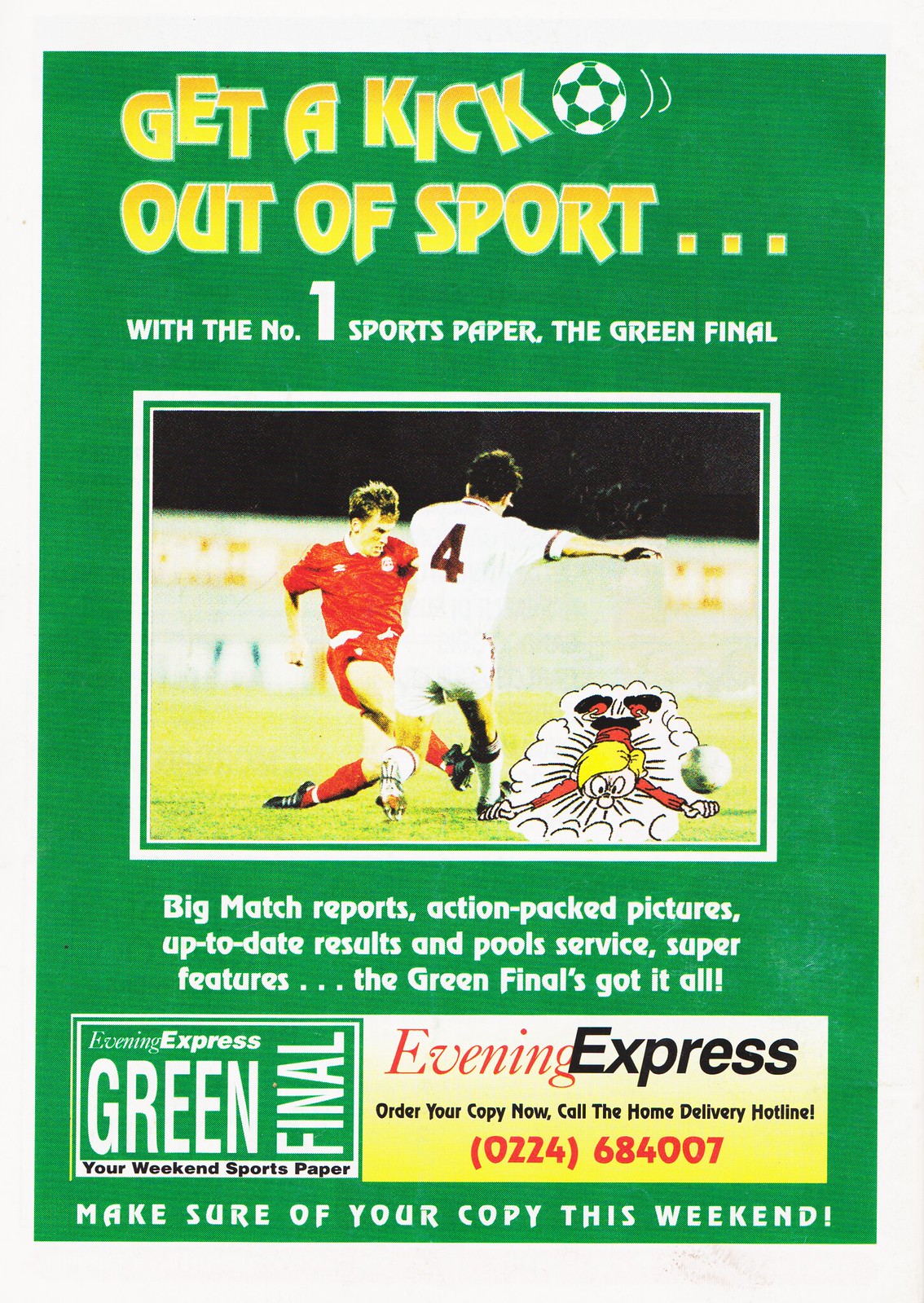The magazine cover has a vibrant green background with eye-catching yellow lettering at the top that reads, "Get a Kick Out of Sport." The word "kick" is stylized with the final "k" slanting to nudge a small soccer ball graphic. Below this is the slogan "with the number one sports paper, The Green Final," in bold white text. 

Dominating the center of the cover is a dynamic photo of two professional soccer players, one in a red jersey and the other in a white jersey, vying for the ball on the field. Overlaid on the image is a playful cartoon of a character with yellow hair sliding toward the camera.

Beneath the photo, a rectangle contains text promoting the magazine's offerings: "Big match reports, action-packed pictures, up-to-date results, pool service, super features—the Green Final's got it all." At the very bottom, the logo "Evening Express Green Final: Your Weekend Sports Paper" appears, along with an urgent call to action: "Order your copy now! Call the home delivery hotline 0224 684007. Make sure you get your copy this weekend." 

The cover is designed to instantly capture the reader's attention with its energetic visuals and promise of comprehensive sports coverage.